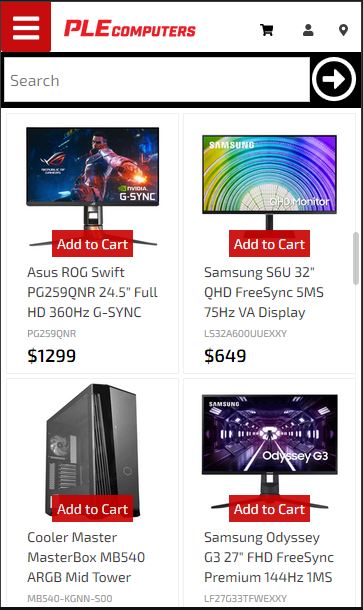This is a detailed descriptive caption for the mobile app screenshot mentioned:

---

The mobile app screenshot features a navigational header at the top. In the top left corner, there is a red square icon with three white horizontal lines, likely indicating the settings menu. Next to this icon, the company name "PLE COMPUTERS" is prominently displayed in uppercase red font against a white background. Adjacent to the company name, from left to right, are icons for a shopping cart, user profile, and location. 

Directly below the header is a white search field with a circular, right-facing arrow icon on its right for initiating searches. 

The main content area showcases four purchasable items in a grid format:

1. **Asus ROG Swift PG259QNR** – A 24.5-inch Full HD monitor with a 360Hz refresh rate and G-Sync technology, priced at $1,299.
2. **Samsung S6U** – A QHD monitor, model S6U, featuring a 32-inch display, FreeSync technology, 5ms response time, and 75Hz VA panel, priced at $649.
3. **Cooler Master MasterBox MB540** – An ARGB mid-tower case designed for PC builders.
4. **Samsung Odyssey G3** – A 27-inch Full HD monitor with FreeSync Premium, 144Hz refresh rate, and 1ms response time.